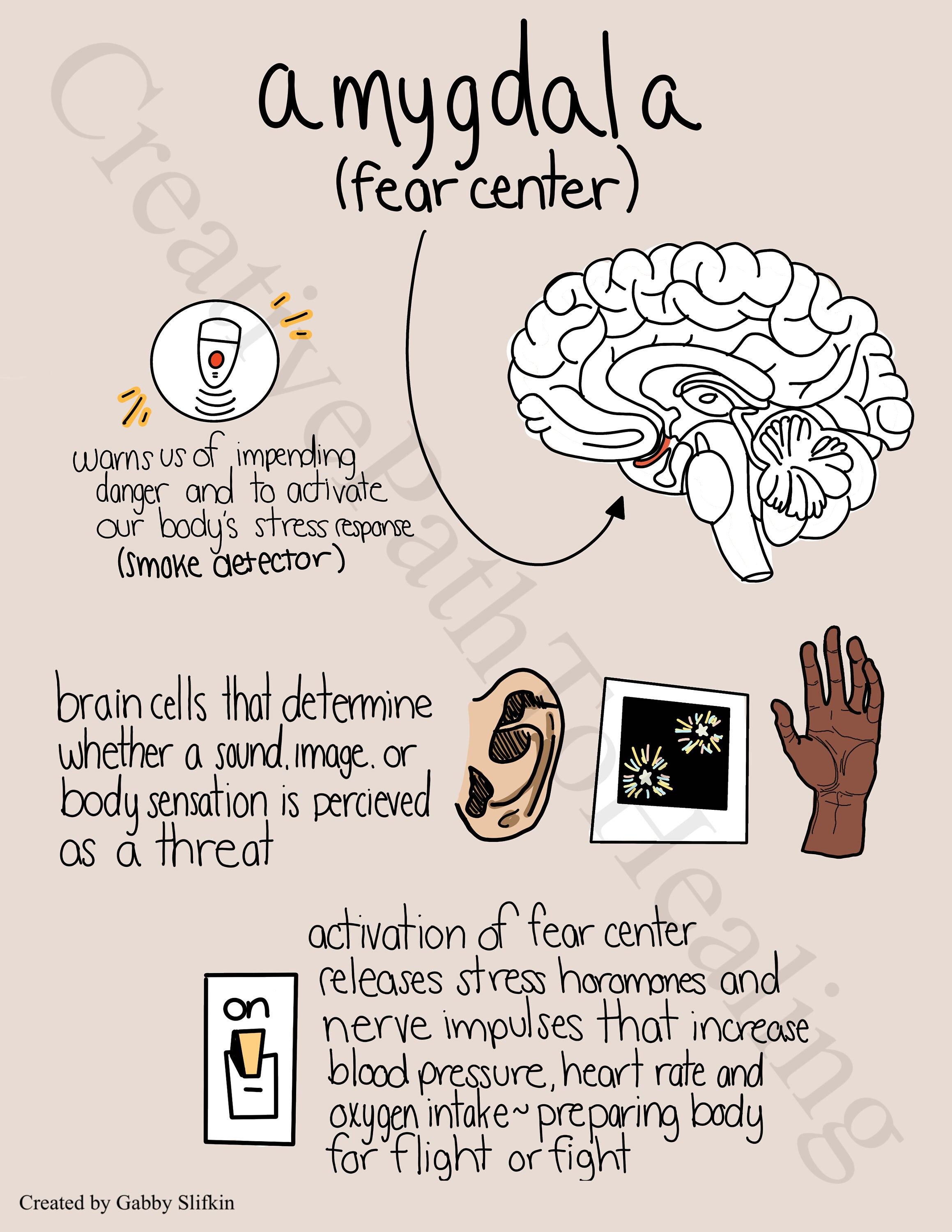The vertical, portrait-style chart titled "Amygdala (Fear Center)" designed by Gabby Slifkin features a detailed cartoon-style illustration and text. It contains an arrow pointing to a labeled black and white picture of the brain, highlighting the amygdala. To the left, an icon resembling a mouse in a white circle notes, "Warns us of impending danger and to activate our body's stress response," with "smoke detector" in parentheses. Below, it states, "Brain cells that determine whether a sound, image, or body sensation is perceived as a threat." To the right of this text, there's an illustration of an ear, stars, and a raised hand. Further down, the chart explains, "Activation of fear center releases stress hormones and nerve impulses that increase blood pressure, heart rate, and oxygen intake, preparing the body for fight or flight," accompanied by a drawing of a light switch turned on. A watermark across the page reads, "Creative Path to Healing."